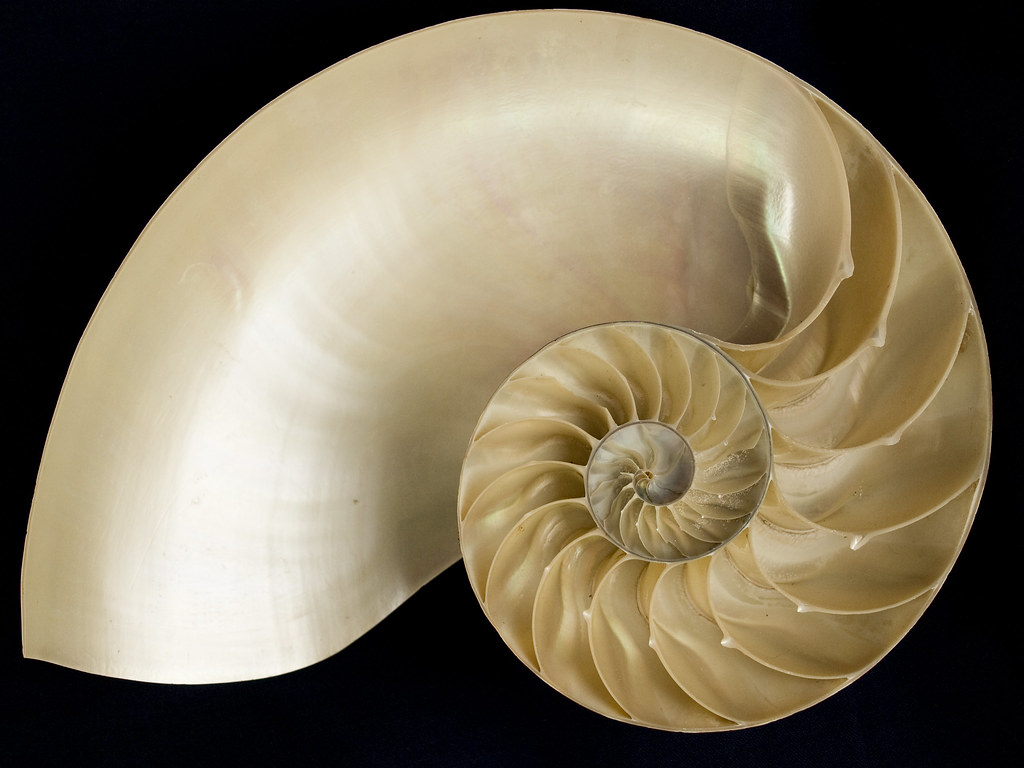The photograph showcases the intricate interior of a nautilus shell that has been precisely sliced in half, revealing its mesmerizing internal structure. The shell, displayed against a pitch-black background, is a light yellowish tan with a subtle pearlescent sheen that adds a touch of elegance to its appearance. The nautilus shell curves gracefully into an almost perfect semicircle before spiraling inward approximately two and a half times, becoming progressively smaller towards the center. The left side of the shell's exterior is perfectly smooth and devoid of texture. Inside, a series of small, fan-like ridges follow the spiral's curve, creating a satisfying yet non-symmetrical composition that is both visually captivating and geometrically fascinating.